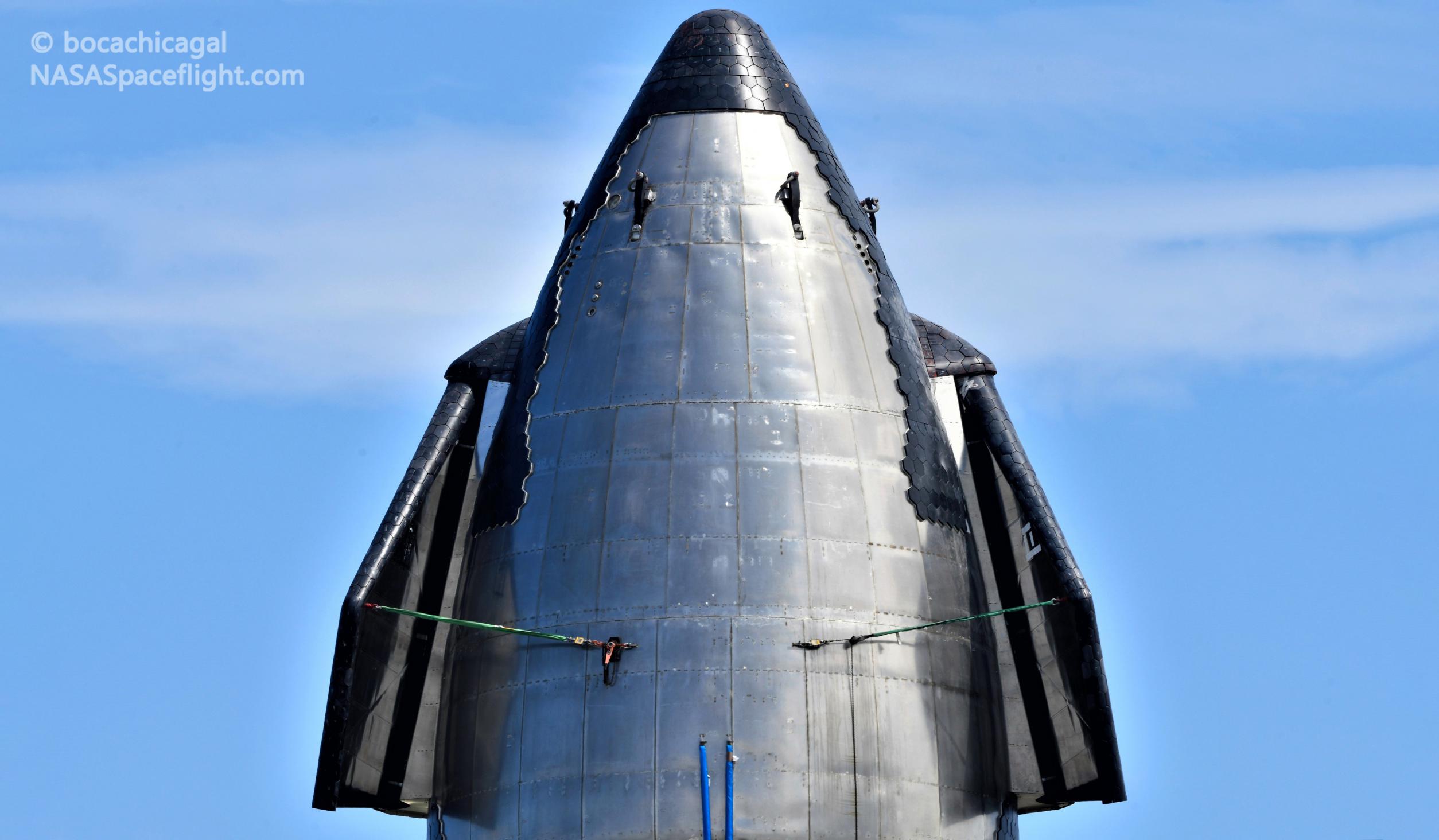This captivating image, sourced from nasaspaceflight.com and credited to Boca Chica Gal, features the upper section of a NASA rocket set against a clear, light blue sky with a scattering of wispy white clouds. The sleek, silver rocket stands prominently at the center of the frame, its nose cone outlined in striking black. Below the nose, black wing-like structures protrude from the body, highlighted by silver and infused with some green cords. The rocket is further framed by associated structures, including a black metallic platform to the side and two distinctive blue rods at the base of the image. The image showcases fine details, such as the silver grid-like patterns on the rocket's surface and various lines leading to it, emphasizing the technical intricacies of spaceflight. The photograph includes a watermark in the top left corner featuring the text "Boca Chica Gal" and "nasaspaceflight.com," acknowledging the photographer.